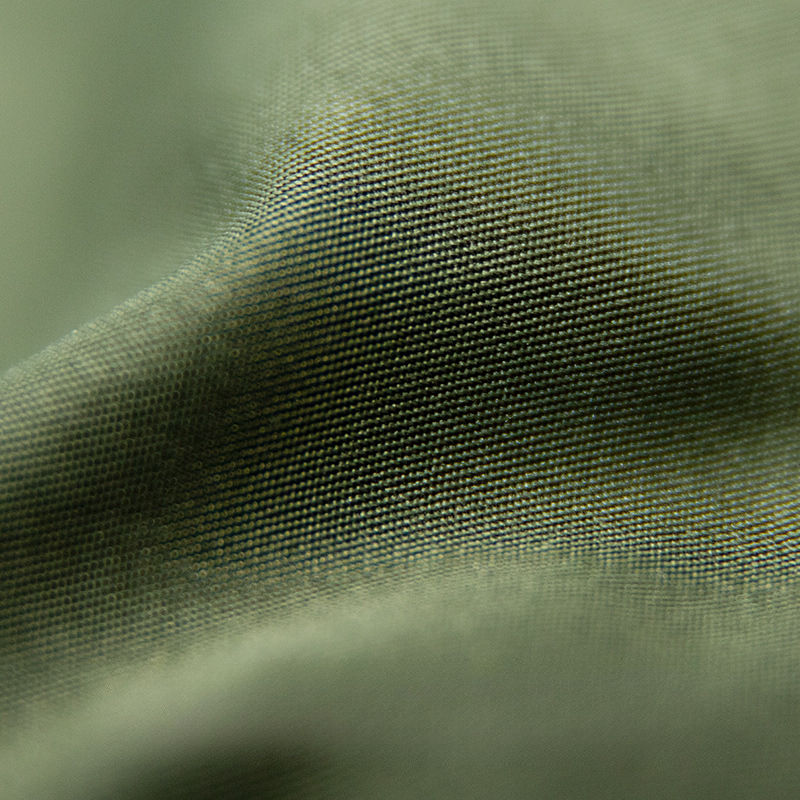This is a highly detailed close-up color photograph of a piece of fabric, capturing its intricate texture and subtle color variations. The fabric appears to be a greenish-gray color, with sage green highlights and darker, more forest-green shadows, although both colors are muted and grayish. The material is tightly woven, evident from the hundreds of small threads that can be seen clearly in the focused center of the image. The bottom front and top edges of the photo are out of focus, which emphasizes the texture and depth in the central area. A noticeable wave-like fold runs vertically through the middle of the fabric, producing a shadowy "canyon" that contrasts with the lighter, more illuminated edges. Despite the thickness suggested by its texture, the fabric bends gracefully, hinting at its flexibility. No additional colors or text are present in the image.